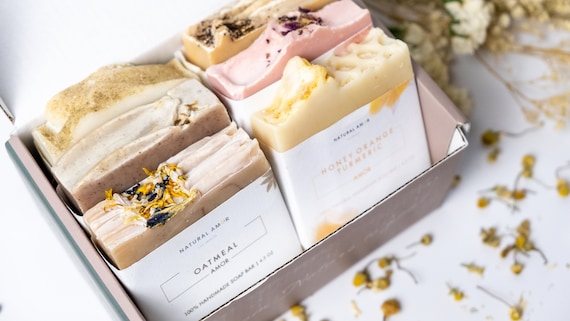The photograph features a small cardboard box filled with artisanal soap bars, set on a white table sprinkled with small crushed leaves and dried flower petals. The box, viewed from an aerial angle, has its lid open to reveal two neatly arranged rows of soap, each containing three bars. The front left soap is a brown-topped oatmeal soap with a sprinkling of dried flowers, while the soap next to it is light beige, labeled as honey orange turmeric soap. Although the exact labels of the soaps in the background rows are unreadable, the soaps appear to be of various natural colors, including yellow and pink. Each soap bar has a white label with predominantly black writing, and some of the labels include descriptive phrases such as "100% handmade soap bar" and "natural." The overall presentation suggests these soaps are handcrafted and possibly organic, with an aesthetic that could easily be mistaken for artisanal desserts.